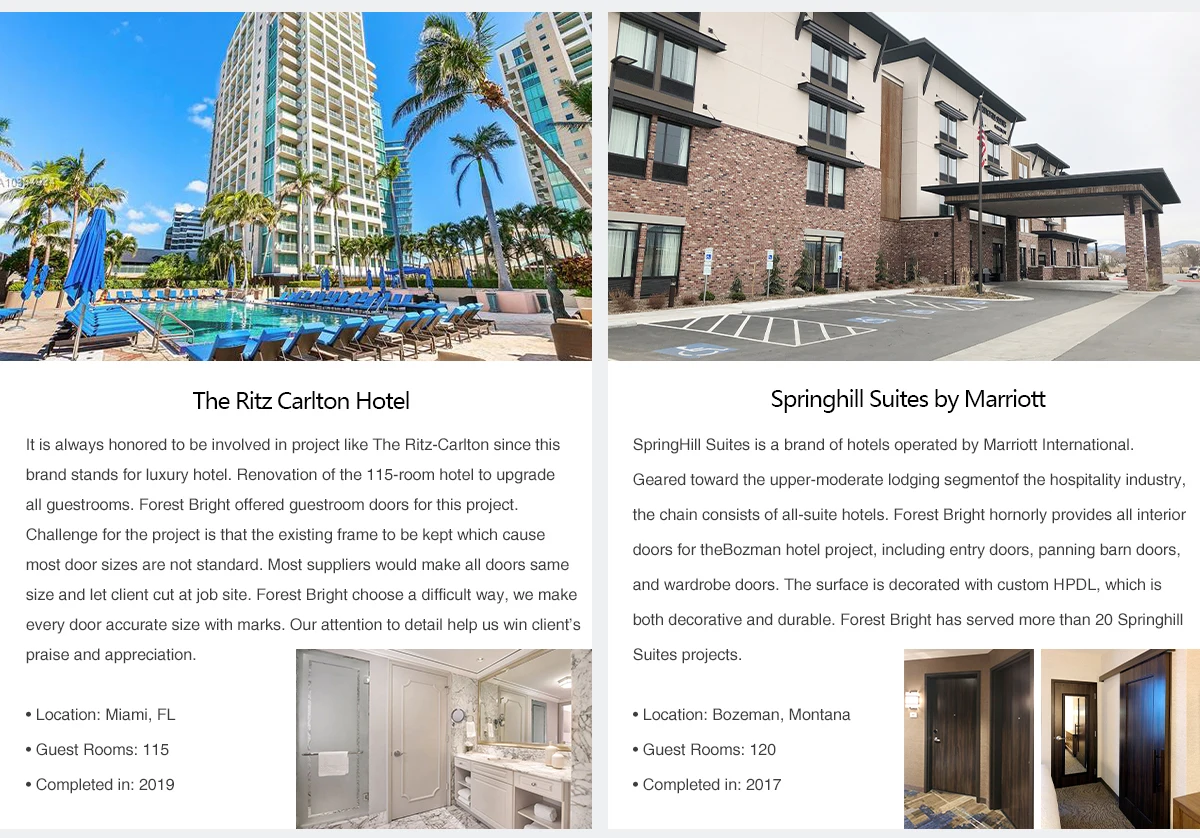In this image, we can see a picturesque scene highlighting two prominent hotels. Dominating the skyline on the left is the luxurious Ritz Carlton Hotel, a symbol of opulence and elegance. The Ritz Carlton is undergoing significant renovations to upgrade all 115 guest rooms, ensuring that the hotel maintains its esteemed standards. Despite challenges such as retaining the existing door frames, Forest Bright has meticulously crafted custom-fitted doors for each room.

To the right side of the image stands the Spring Hill Suites by Marriott, a line of hotels known for catering to the upper-moderate lodging segment. The photograph captures the hotel's signage clearly. The Spring Hill Suites property features comfortable blue chairs and umbrellas by a pool, set against a backdrop of a bright blue sky with scattered clouds and lush palm trees. The asphalt below includes marked lines and designated handicapped parking spaces. Forest Bright has been instrumental in the interior design of multiple Spring Hill Suites projects, providing high-quality interior and wardrobe doors.

Situated in scenic Miami, Florida, the dual-hotel view encapsulates a harmonious blend of luxury and comfort, with the Spring Hill Suites completing its latest project in 2019. The attention to detail and customized solutions offered by Forest Bright underscore the image, reflecting their commitment to excellence in hospitality design.